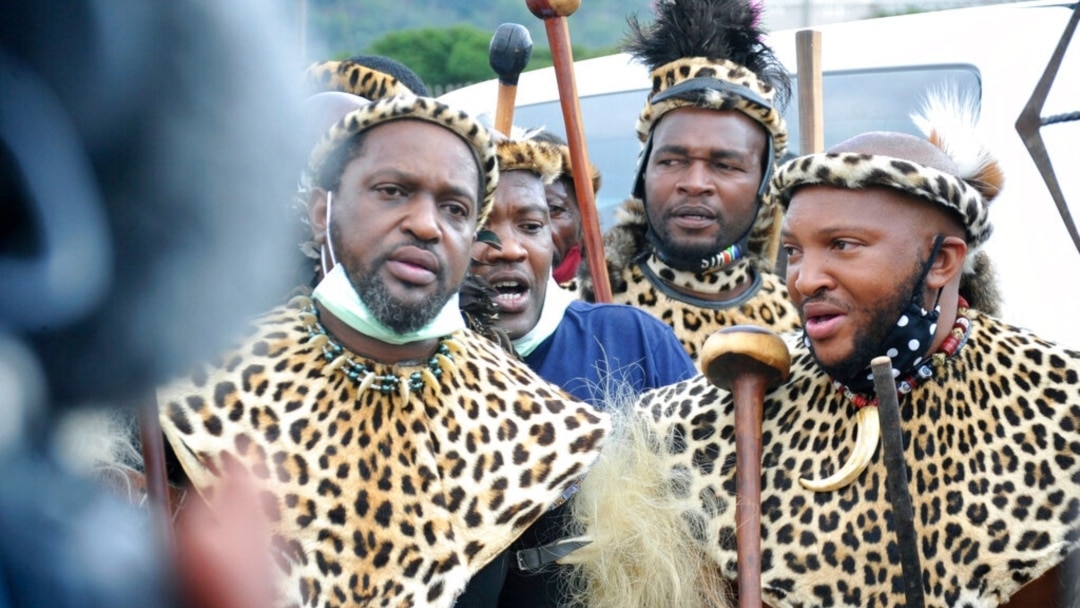The image depicts a group of African-American men standing closely together outdoors in daylight, adorned in elaborate tribal attire. Each man is wearing a distinctive cheetah or leopard-print garment that drapes over their heads, chests, and backs. Complementing their outfits, they have on vibrant, colorful beaded necklaces, some decorated with what appear to be animal teeth. Their heads are adorned with headbands of the same cheetah fabric, each tucked with various feathers, enhancing their ceremonial appearance. The men are bearded and clutch long wooden sticks with round spear tips, seemingly in the midst of singing or chanting. Notably, one gentleman stands out as he is dressed in a blue t-shirt instead of the customary cheetah garb. The background features a blurred dark figure on the right side and a white band with a window exhibiting a V design. The scene is set against a backdrop of foliage under the bright sunlight.